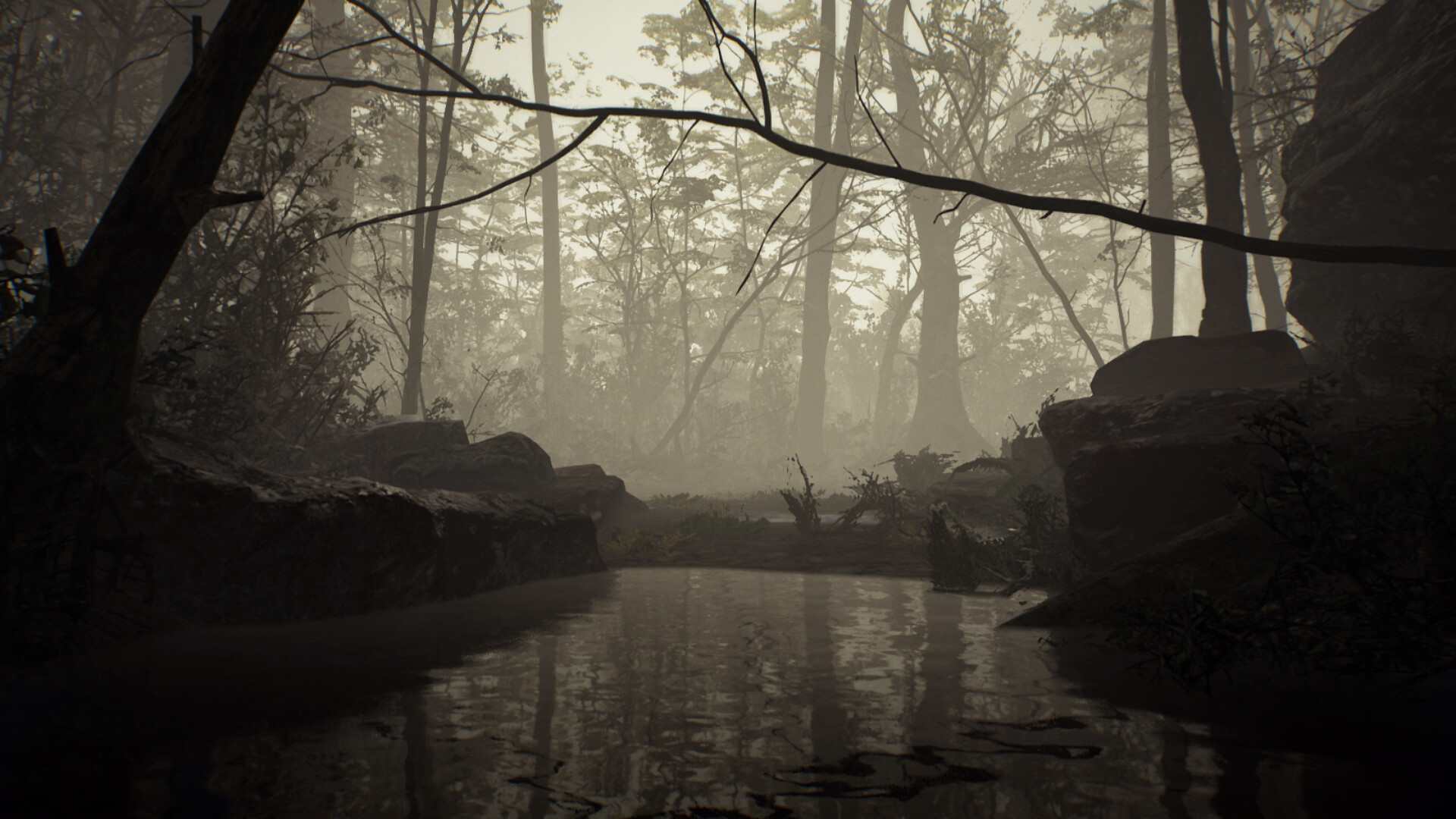A hauntingly beautiful black and white photograph captures a small, serene pond surrounded by smooth, picturesque rocks and delicate ferns emerging from the water's edge. The grayscale tones contribute to the eerie yet enchanting atmosphere, with myriad shades of gray enhancing the photograph's depth and complexity. In the background, a foggy, wooded area stretches out, with the silhouette of thin tree limbs and smaller trees forming an intricate lattice. The mist diffuses the light, creating the impression of a distant, ethereal sunset that adds a soft, glowing quality to the scene. The overall composition merges the tranquility of nature with an unsettling, almost mysterious ambiance.